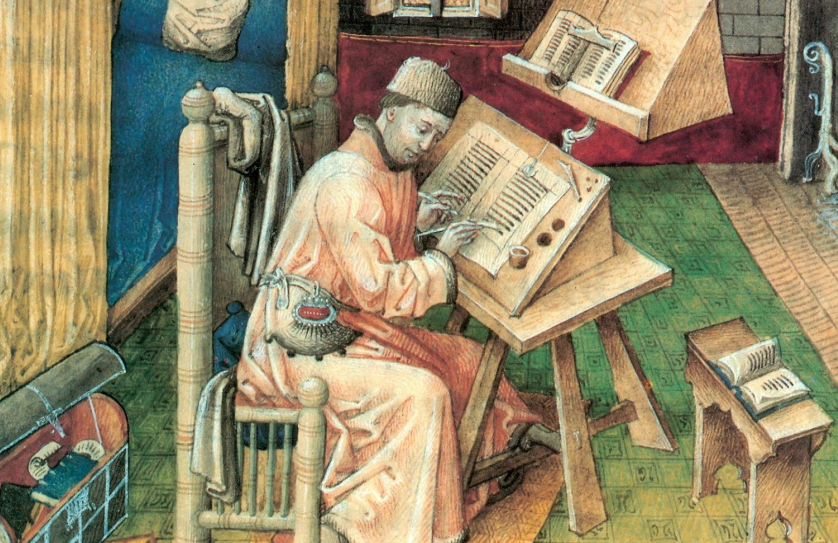This painting, reminiscent of the medieval era, depicts a scribe or monk meticulously copying a manuscript. The setting, suggesting a timeframe between the 12th and 13th centuries, showcases the subject seated at a wooden desk. The scribe, dressed in a long, peach-colored robe and a simple hat, is engaged in writing with a quill on large sheets of paper. To his right, an easel supports a smaller reference book, while an inkpot is placed nearby on the table. The room features a greenish-bluish tiled floor accompanied by red and blue trims on the walls, typical of medieval artistic perspective where the depth perception is noticeably primitive. Behind the scribe, there's a chest filled with various indistinct items, hinting at a cluttered yet scholarly environment. The scribe also has a satchel fastened to his side, reinforcing the scholarly or monastic nature of his work.